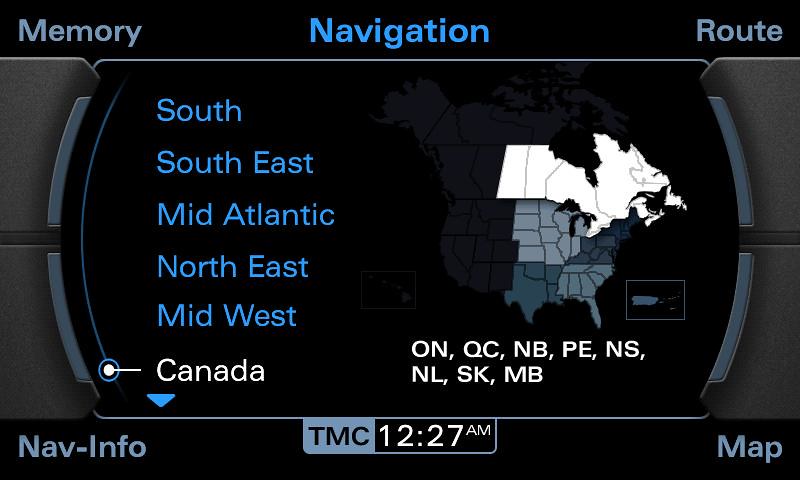The image is a rectangular navigation screen with a predominantly black background, accented with shades of gray, light blue, and white lettering. The top left corner features the word "Memory" in gray, while the center highlights "Navigation" in light blue and the top right corner displays "Route" in gray. Below this header lies a list of regions aligned along the left side in blue text: South, Southeast, Mid-Atlantic, Northeast, Midwest, and Canada, with Canada highlighted by a white dash. To the right, a detailed map of the eastern half of the United States and Canada is displayed, with Canada brightly lit in white, contrasting against the grays and blues of the United States. The map provides a clear visualization of specific states and provinces, including ONQC, NB, PE, NS, NL, SK, and MB. The bottom of the screen includes "Nav-Info" on the left, "TMC" and the time "12:27 AM" positioned centrally, and the word "Map" in the lower right corner. The image has rounded gray side panels framing the central display area.